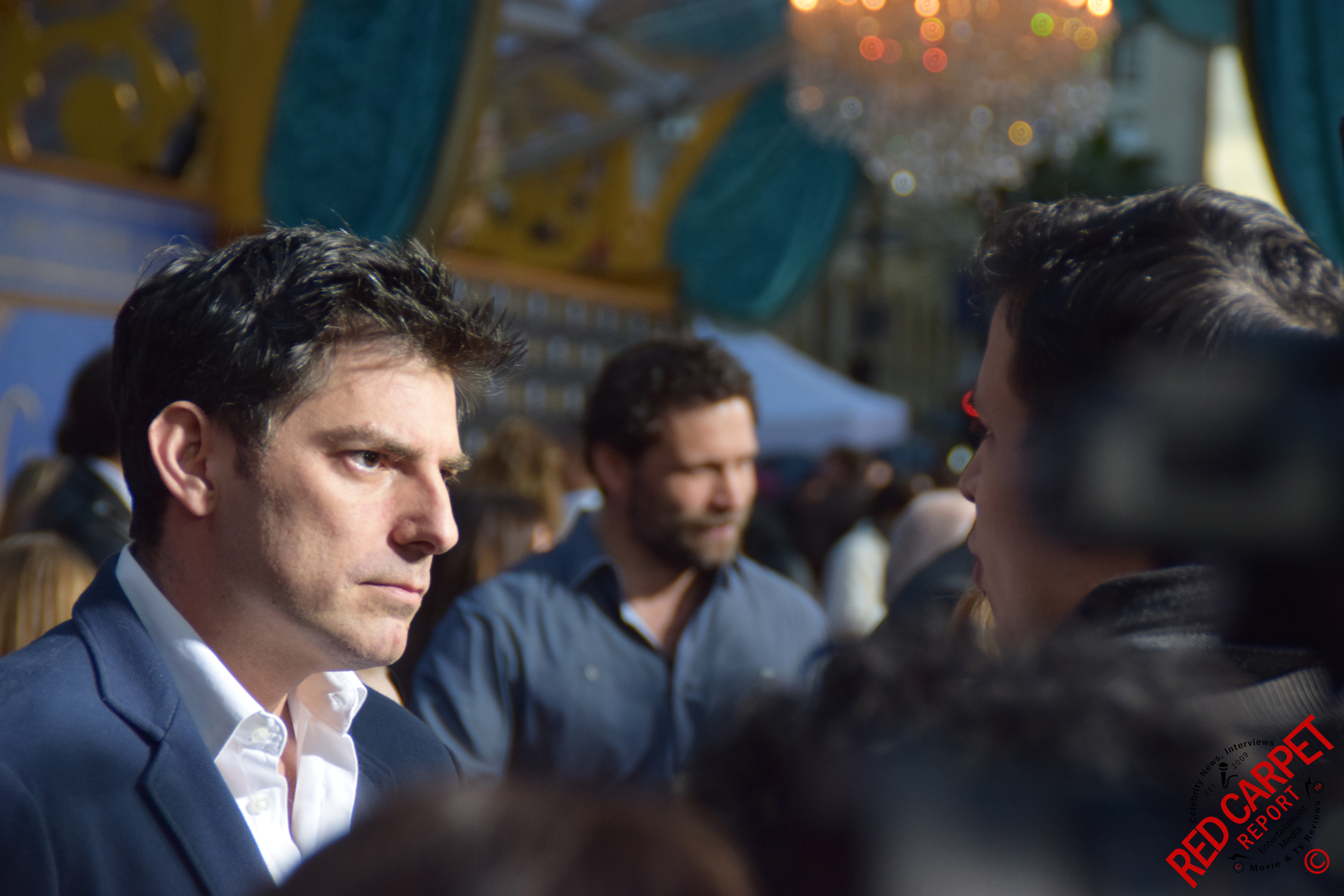In the photograph captured at a glamorous indoor event, possibly a red carpet gathering, a crowd of people with many out of focus fills the background. The primary focus is on a clean-shaven man on the left side of the image with gelled, dark brown hair, spiked at the front. He is wearing a blue suit with a white button-up shirt and exhibits a stern expression as he intently listens to another man on the right side. This man, whose face is partially visible with his mouth appearing slightly open, also has short black hair and is clad in a black collared shirt. Between them, and slightly blurred, stands another man with curly brown hair, a beard, and a blue shirt, appearing to smile and look off to the right.

A polished chandelier hangs prominently in the upper central part of the image, its reflections contributing to the sophisticated ambiance of the room, which features high arched ceilings adorned with blue and yellow tones. Overlaying the bottom right corner of the image, there is a watermark in red capital letters that states "Red Carpet Report" at a 45-degree angle, accompanied by a small 'C' in a circle beneath it.